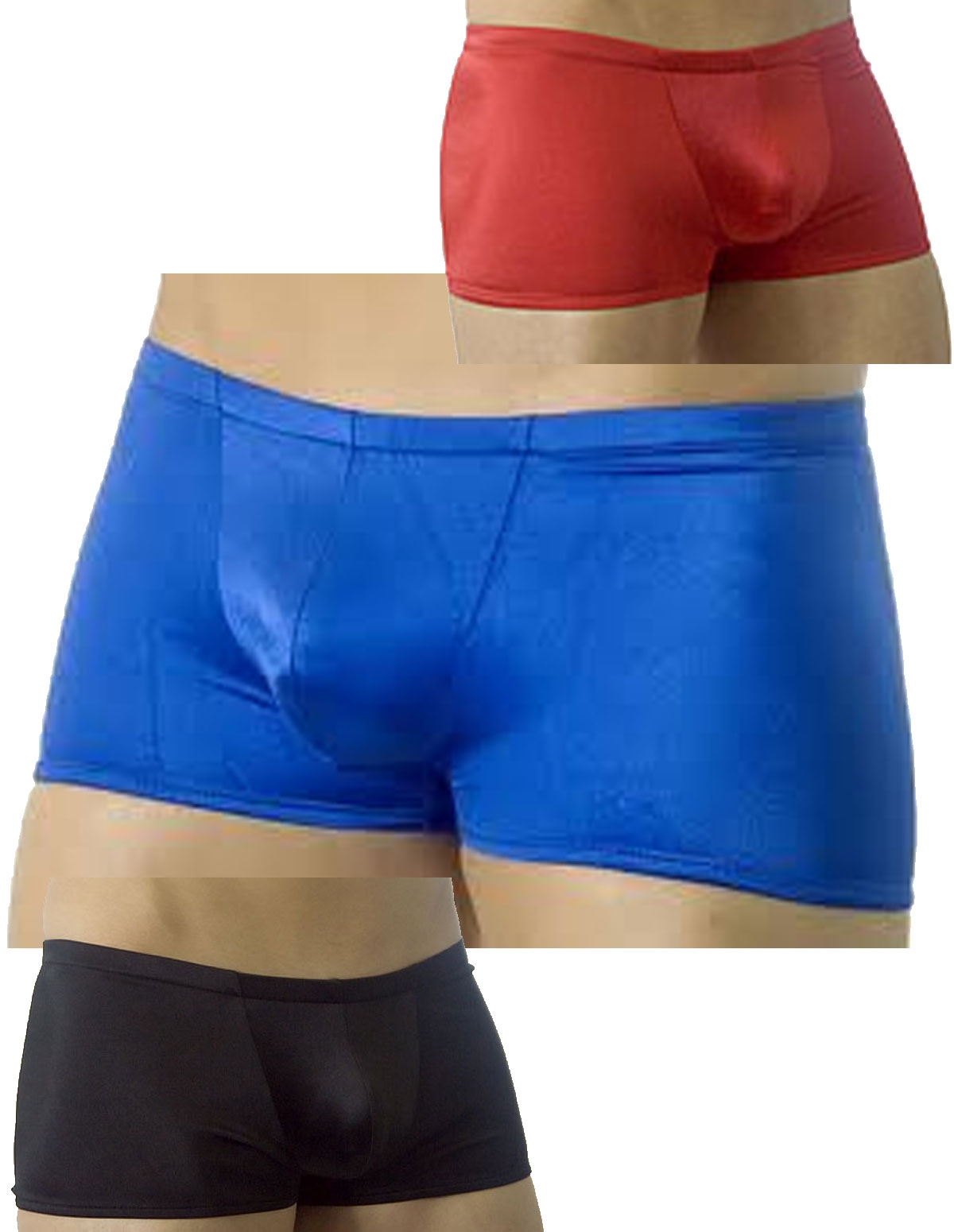This image features a professionally-taken series of three superimposed photos of men's silky, satiny boxer briefs. The composition includes distinct images showcasing the underwear in different colors: a smaller red pair in the upper right quadrant, a larger primary image in bright blue prominently placed at the center, and another smaller pair in black situated in the lower left quadrant. The boxer briefs are modeled on a male figure, accentuated by a noticeable bulge that adds an element of awkwardness. The background is pure white with no text, logos, or visible branding. The only colors present in the image are black, white, red, blue, and the tan skin tone of the model. The professional photography suggests it could be sourced from either a clothing website or an adult site.